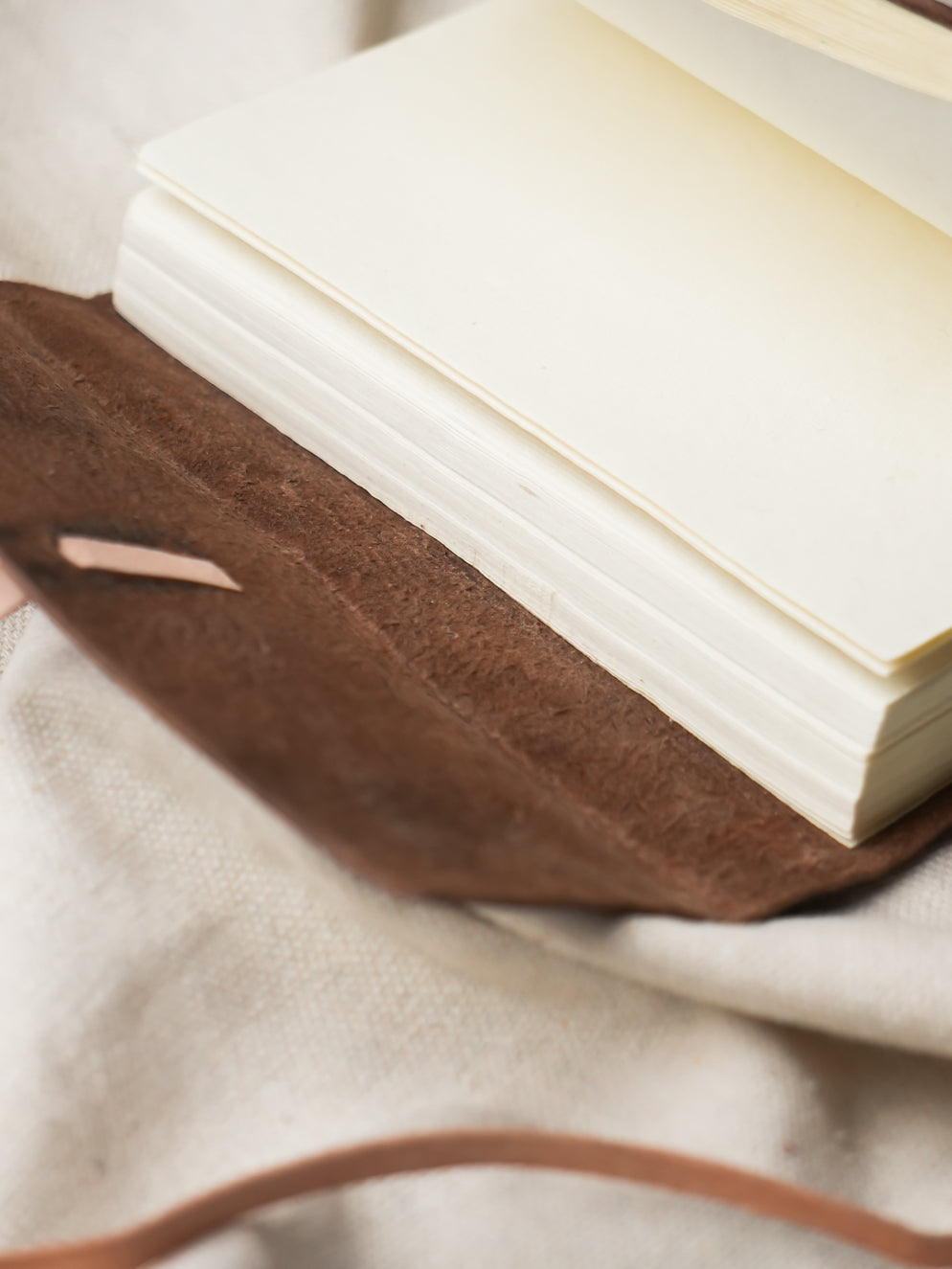The image features an elegant scene centered around an empty journal resting atop luxurious fabric. The journal, bound in a supple brown leather casing, has a pale salmon tie to fasten it. The many pages, graded from a dark cream to a light cream near the edges, exude a sense of high quality. The journal lies open, causing some of its pages to be concealed on the right side, hinting at its substantial volume. The backdrop is composed of a creamy, gradiated cloth with subtle gray accents, folded in a luxuriously decadent manner. The overall composition, with its blend of rich browns and creamy hues, evokes a refined and cozy atmosphere.